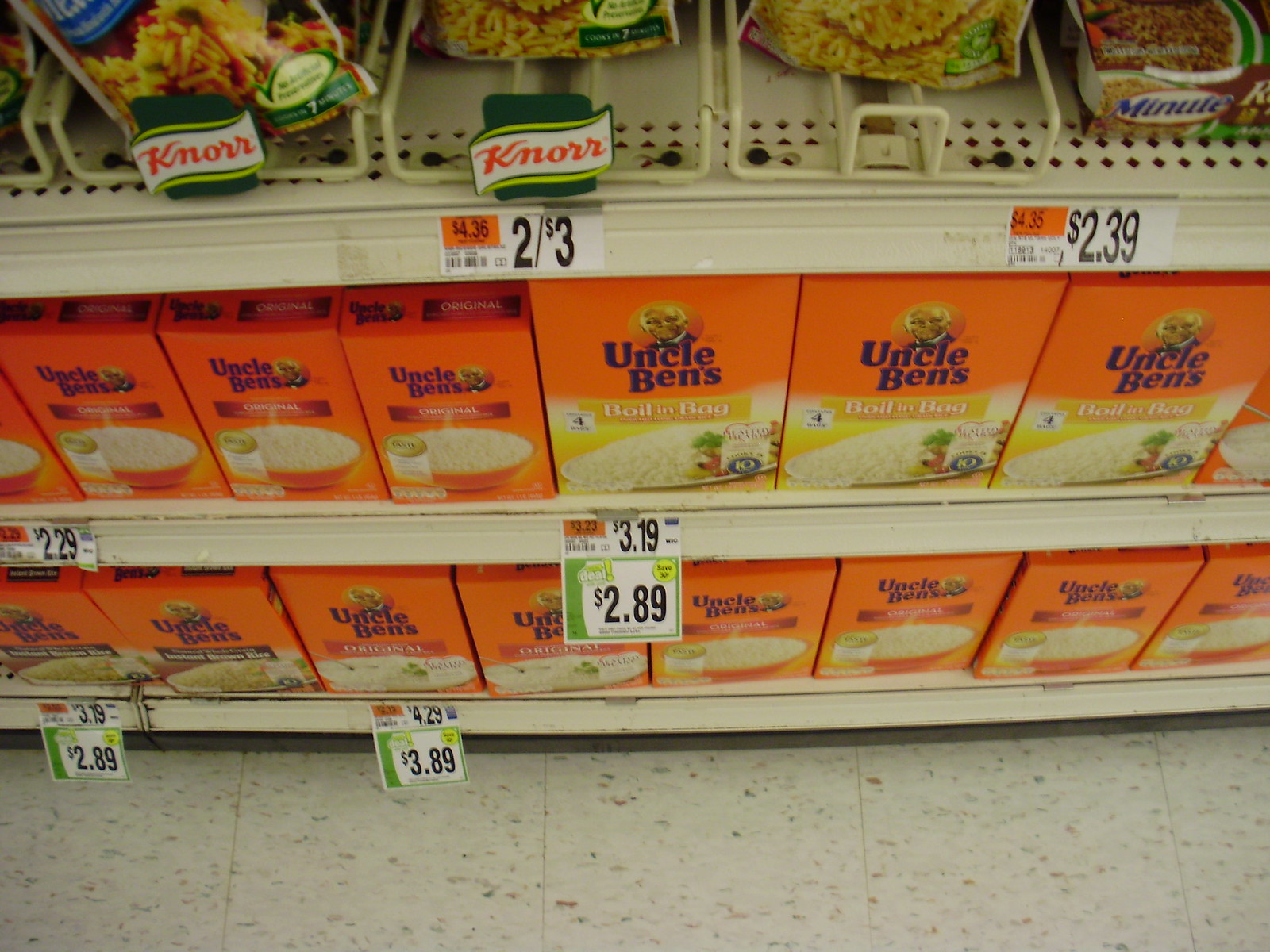This image, taken from a downward angle inside a grocery store, highlights three shelves stocked with food products. The bottom shelf features a cream-colored floor beneath a tan steel-edged rack adorned with green and white price stickers. This entire shelf is filled with Uncle Ben's rice products, including original and boil-in-bag varieties, with prices such as $2.29, $3.19, and a promotional price of $2.89. The middle shelf continues the display of Uncle Ben's products, showing different sizes. The topmost shelf displays an array of Knorr pasta packets organized in five sections, with prices around $2 to $3 per item. Additionally, the right side of the image includes Minute Maid ready rice priced at $2.39.